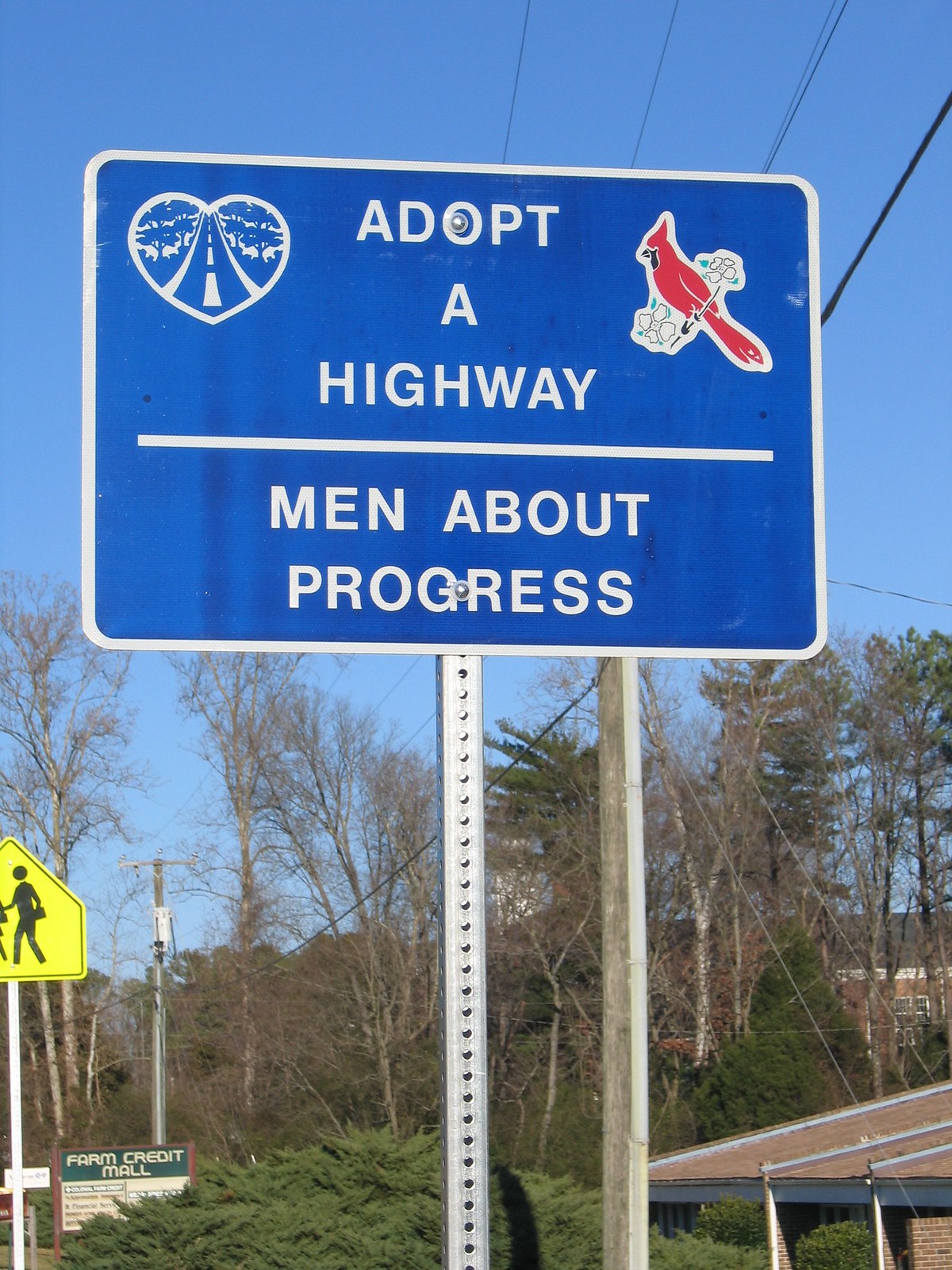The image depicts a blue highway sign, prominently positioned along the roadside, designated as an "Adopt a Highway" sign. The sign features white text and illustrations: on the left side, a heart with a stylized road and dashed lines inside, and on the right side, a red cardinal bird. Below the main text, a horizontal line separates it from the label "Men About Progress," indicating that this group has committed to maintaining this stretch of road.

Surrounding the sign, the background reveals a clear blue sky dotted with trees. To the right, the roof of a house is slightly visible, while to the left, a partially visible yellow crosswalk sign, shaped like a house with child pedestrian icons, can be seen. In the distance, there appears a structure or advertisement labeled “Farm Credit Mall,” further enhancing the suburban setting. The scene overall captures a community-driven effort to keep the local environment clean and well-maintained.